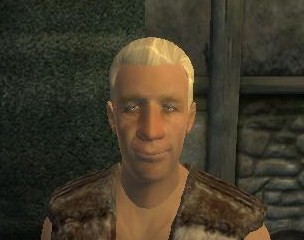The image is a small 2x2-inch screenshot captured from the video game "The Elder Scrolls: Oblivion." It features a highly detailed 3D character, an older gentleman with glossy gray or white hair that appears shinier on the right side and more matte on the left, suggesting a light source from that direction. The man has a large nose, narrow, almost sleepy eyes, and a closed mouth with a mild, non-grinning smile, giving him a serene expression. He dons a vest made from animal pelt, likely a caveman-type design, over a faded pink shirt. Behind him, the background showcases a rustic interior with stone walls and wooden beams, possibly hinting at an ancient or primitive setting. Notably, the left side of the wall features a green design, while the right side hints at a caveman-like rock formation or structure.